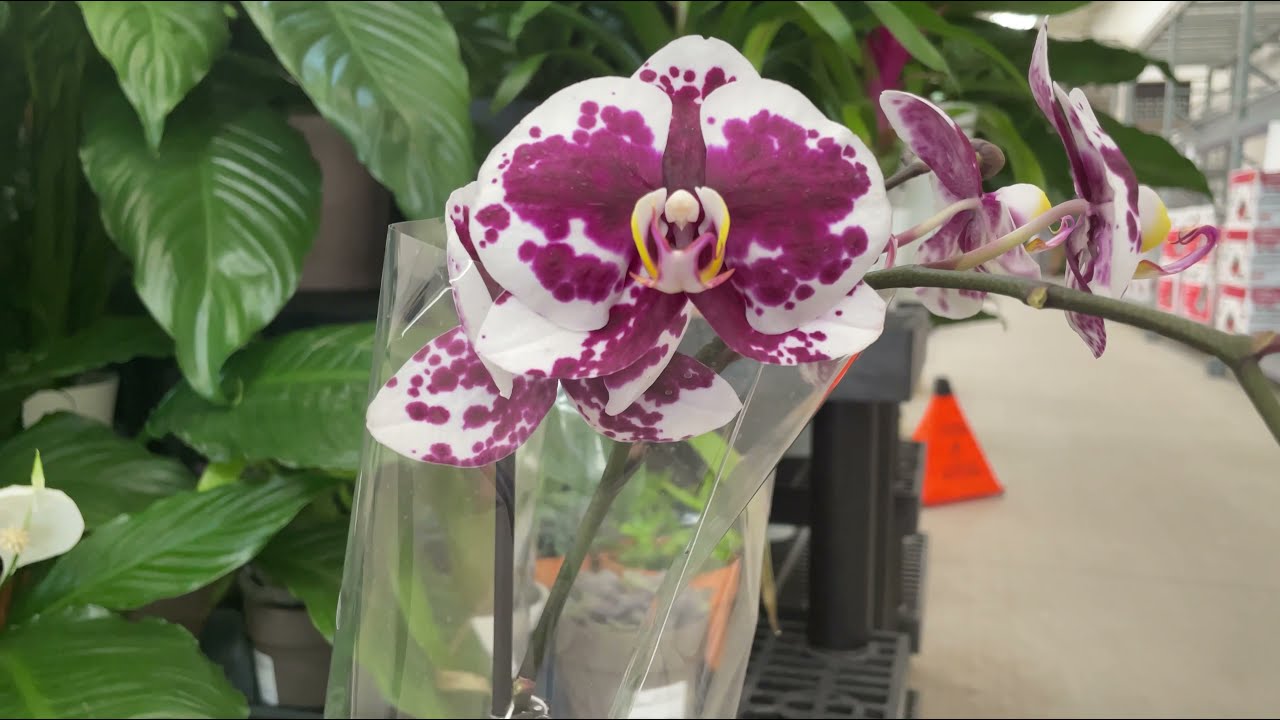This photograph depicts a close-up view of a maroon and white orchid flower, perfectly highlighted by its intricate petals that boast a captivating speckled pattern reminiscent of blood spatter. The flower's vivid yellow pistil stands out at the center, resembling a mouth-like shape from the Predator movie. The bloom is supported by a thick green stem, which is secured to a black bamboo stick and encased in cellophane plastic, suggesting it's ready for sale. The scene is set within a store or a department warehouse, evidenced by the metal shelves and a mix of red-and-white cardboard boxes stacked behind the flower. Additional plants, characterized by lush green leaves in cheaper-looking plastic pots, populate the background. The floor beneath is made of concrete, with a noticeable yellow caution cone placed in the walkway, presumably to warn customers of potential hazards.